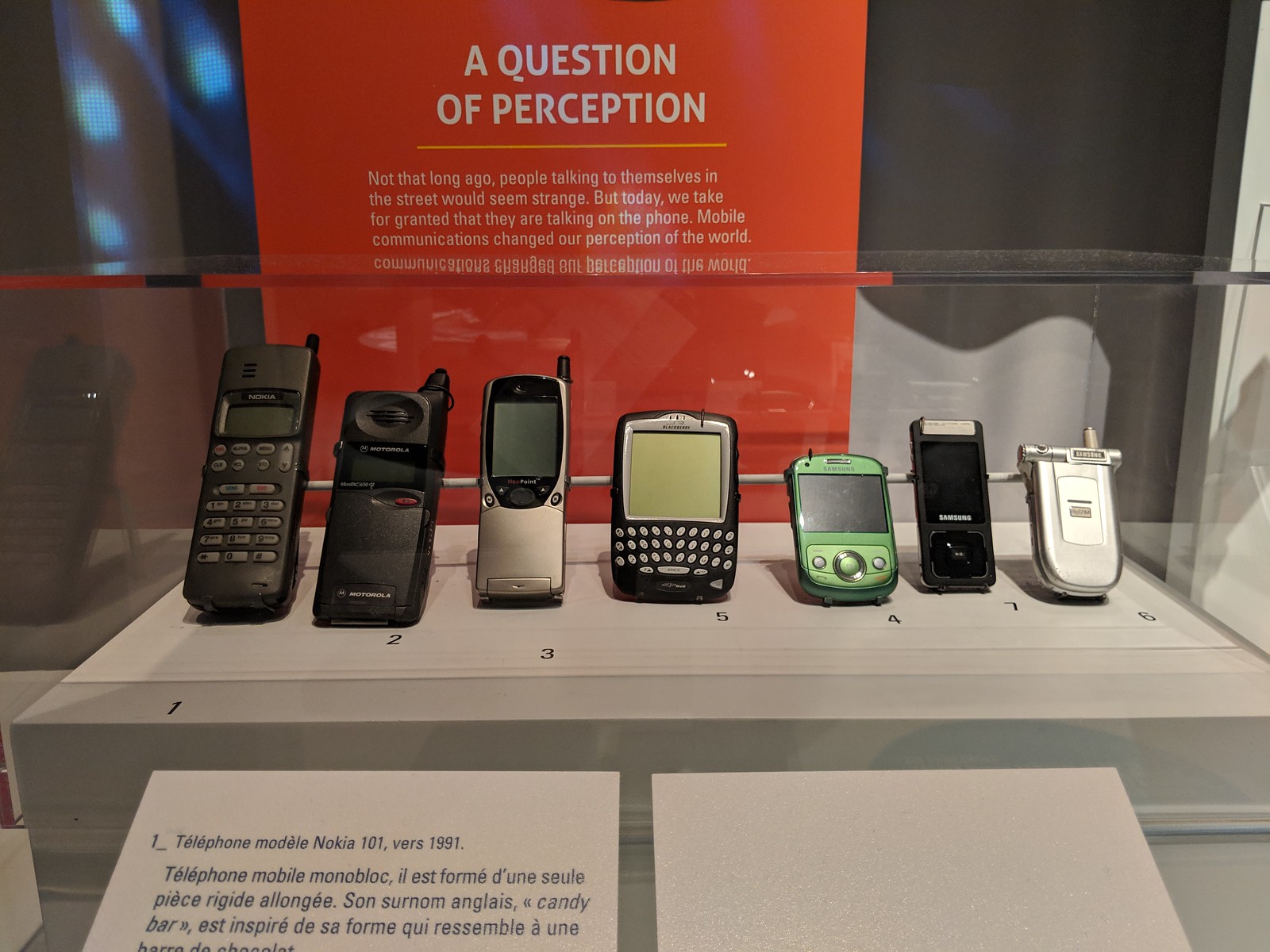The photograph depicts a glass display case housing seven retro mobile phones, arranged in a left-to-right gradient from older, larger models to newer, smaller ones. Starting from the left, there are several black phones, including one with buttons reminiscent of the 1990s, and another that appears to be a Nokia model from the early 2000s with a larger screen and a button cover. Centrally placed is a BlackBerry with a full QWERTY keyboard. Further to the right, a luminous green phone catches the eye due to its unique color and minimalist design with just three buttons at the bottom. The final phone on the right is a silver flip phone, marking the shift towards more compact, portable designs.

Behind the display, a red poster with white text poses the question "A Question of Perception." Underlined in orange, the text below reads, "Not that long ago, people talking to themselves in the street would seem strange, but today we take for granted that they are talking on the phone. Mobile communications changed our perception of the world." Reflections of this text can be seen on the glass case. Below the phones, two white sheets are placed; the one on the left reads "Telephone Model Nokia 101 Version 1991," accompanied by text in a different language, likely a translation into French. The display highlights the evolution of mobile communication technology and the societal changes in its perception.